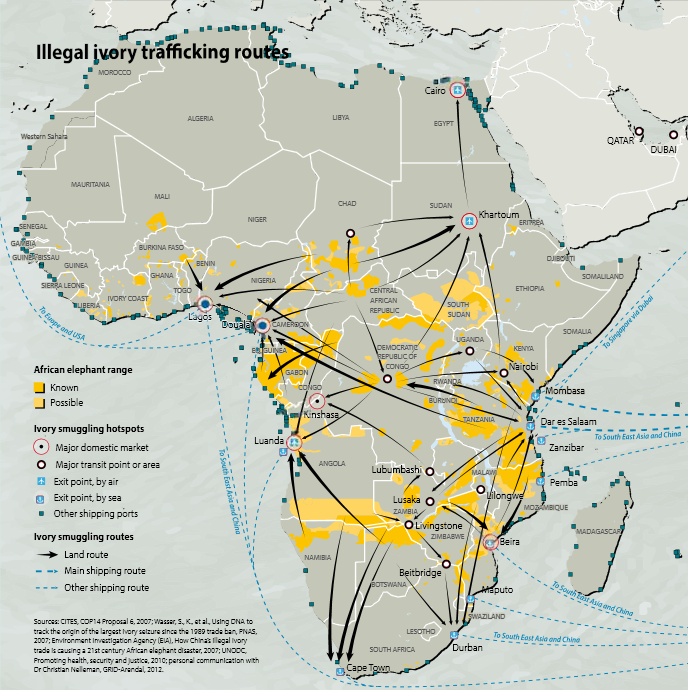This detailed illustration is a shaded map of Africa, rendered in hues of white and gray-blue, depicting "Illegal Ivory Trafficking Routes" in prominent black lettering at the top left. The map extends to include a portion of the Middle East on the upper right. It is extensively annotated with arrows and connection lines illustrating major trafficking routes across the continent. Key cities and regions involved in the illegal ivory trade, such as Chad, Khartoum, Sudan, Tanzania, and Mombasa, are highlighted. 

A detailed legend is positioned on the bottom right, categorizing various aspects of the trade: 
- African Elephant Range: represented in dark yellow for known ranges and light yellow for possible ranges.
- Ivory Smuggling Hotspots: marked with a red circle for major domestic markets, a black circle with a white dot for major transit points or areas, small blue symbols for exit points by air (square with a person inside) and sea (anchor), and dark blue squares for other shipping ports.
- Ivory Smuggling Routes: displayed using black arrows indicating different land routes, with dotted and dashed lines distinguishing main and other shipping routes.

No animals or people are depicted on this map, focusing solely on the trafficking connections and pertinent locations.